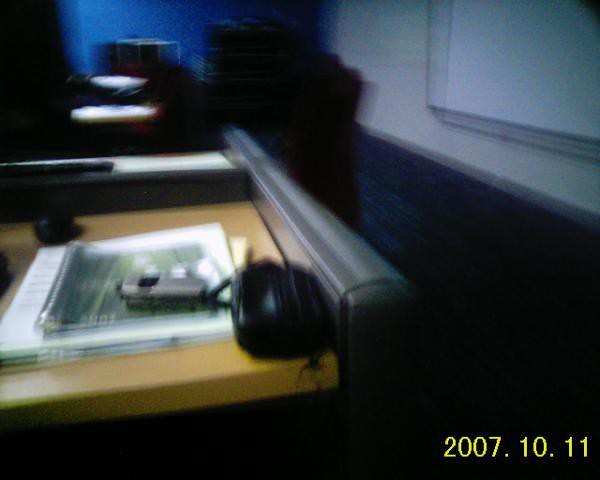This indoor photograph, dated October 11, 2007, showcases a somewhat cluttered desk or work area. The image, albeit blurry, captures the gray corner of a sturdy wooden tabletop. On the left-hand side, various papers and a spiral notebook are scattered across the surface. A black case rests on the desk, with a silver device placed atop the spiral notebook. In the background, black file trays are visible, suggesting an attempt at organization. A whiteboard occupies the right-hand edge of the photo. There's a hint of blue light in the left corner, adding a subtle touch of color to the scene.